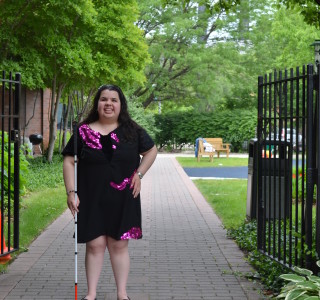This captivating color photograph, set in a square format, features a middle-aged woman standing confidently at the entrance of a picturesque park, framed by an open black wrought iron gate. She stands on the left side of the image, facing the viewer with a warm smile, her left hand resting on her hip. She has long dark hair parted in the middle and appears to be around 40 years old.

The woman is attired in a knee-length, black one-piece duster dress that showcases unique design elements, including purple ruffles adorning one shoulder and the opposite side of the skirt. A distinct pink pocket and coordinating detailing at the bottom of the skirt add further flair to the outfit, likely crafted to feature visually appealing and reflective designs for the visually impaired.

Her right hand firmly grips a white walking stick with a red tip, indicative of the type used by visually impaired individuals. This adds context and depth to her pose, subtly suggesting strength and independence.

She stands on a broad paver walkway that narrows as it extends into the distance, flanked by lush, dark green trees that provide a tranquil backdrop. Behind her, a wooden bench and a Weber grill on a terrace can be spotted, contributing to the scene's outdoor, daytime setting. This detailed and thoughtfully composed image captures not just a moment, but the essence of accessibility and style.